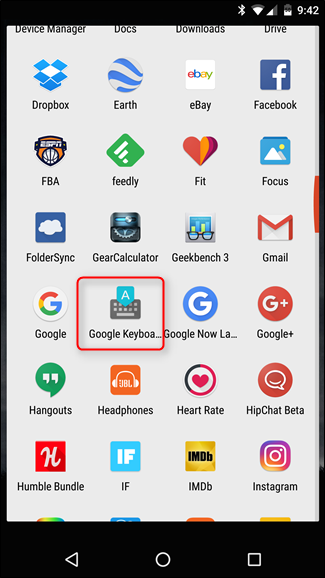The screenshot captures the home screen of an Android phone, focusing on the various applications installed by the user. Key features displayed in the image include:

- **Top Right Corner Details:**
  - **Bluetooth Status:** Activated
  - **Wi-Fi Connection:** Connected with strong signal strength
  - **Cellular Signal:** Approximately two bars
  - **Battery Level:** 50%
  - **Time:** 9:42

- **Applications:** The user's app gallery is extensive and varied, including:

  - **Dropbox**
  - **Google Earth**
  - **eBay**
  - **Facebook**
  - **FBA:** Likely related to basketball, as indicated by the ESPN logo
  - **Feedly:** A green application with a bar graph logo, specific use unspecified
  - **Fit:** Application likely related to fitness, symbolized with a heart icon
  - **Focus**
  - **Folder Sync**
  - **Gear Calculator**
  - **Geekbench 3**
  - **Gmail**
  - **Google**
  - **Google Keyboard:** Highlighted with a red box, indicating it may be of particular importance in this context
  - **Google Now**
  - **Google Plus**
  - **Hangouts**
  - **Headphones**
  - **Heart Rate**
  - **HipChat Beta**
  - **Humble Bumble**
  - **If**
  - **IMDb**
  - **Instagram**

- **Navigation Bar:** Located at the bottom of the screen, featuring:
  - **Back Arrow**
  - **Home Button**
  - **Recent Apps Button** (square icon)

The layout and organization of apps, combined with the phone's status indicators, provide a comprehensive view of the user's Android interface and preferences.